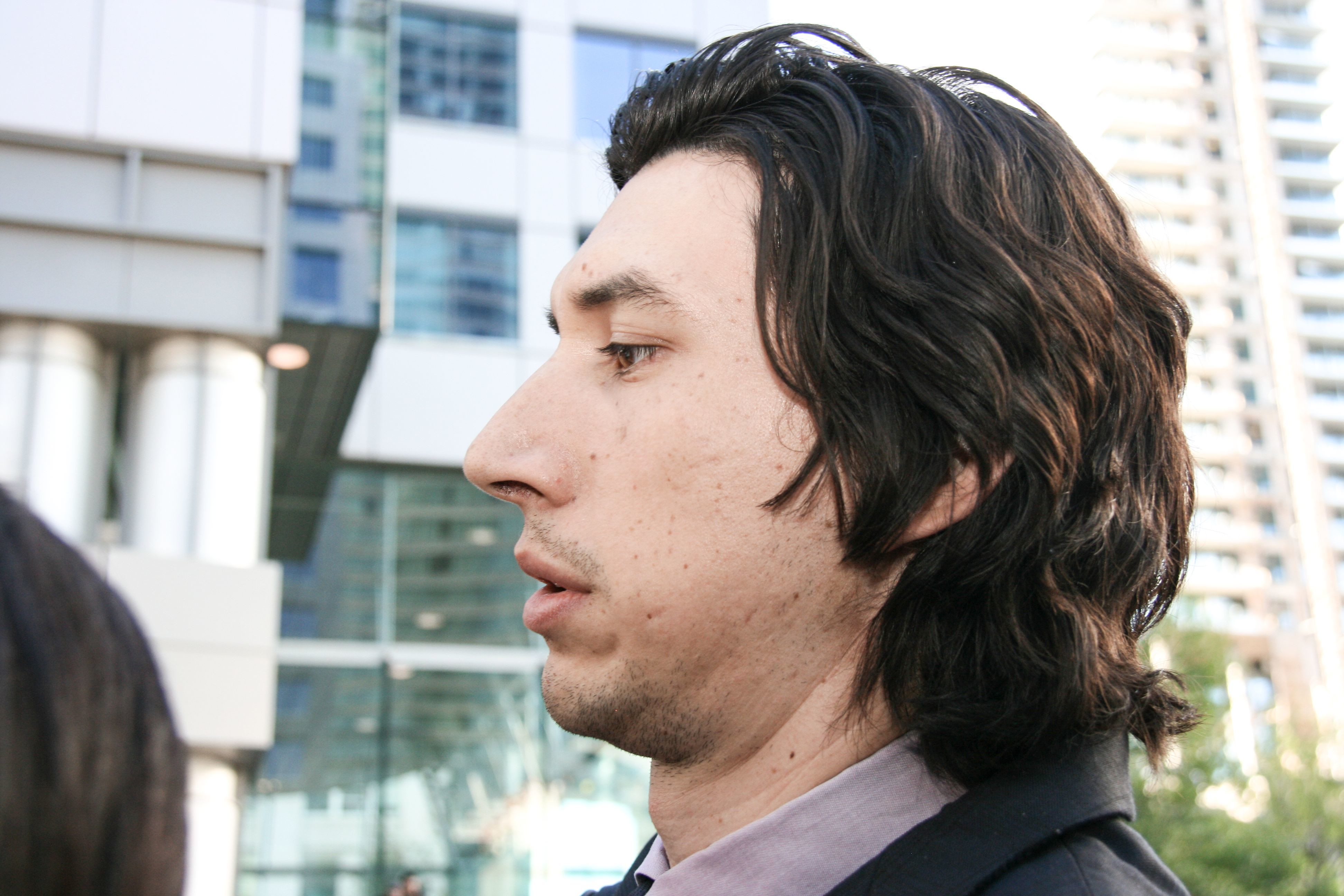This photograph captures a side profile of a man who bears a striking resemblance to the actor Adam Driver, suggesting it might be him. The man has dark brown, wavy hair that extends past his collar, appearing somewhat unkempt and in need of a haircut. His prominent Adam’s apple and long nose stand out, alongside a scruffy mustache and a pronounced five o'clock shadow, indicating he hasn't shaved in a few days. His eyebrows are also unkempt. He is dressed in a black suit coat over a purplish, button-down collared shirt. This individual appears to be in his early 20s and has very pale Caucasian skin. 

He is gazing to the left of the image with a serious expression and a slightly open mouth. Behind him, the background features blurry high-rise buildings, some with more sophisticated, glass exteriors, and others with a cream-colored facade. There are also hints of green leaves at the bottom right corner. In the foreground, on the left side of the image, the blurry outline of another person's head or clothing can be seen.